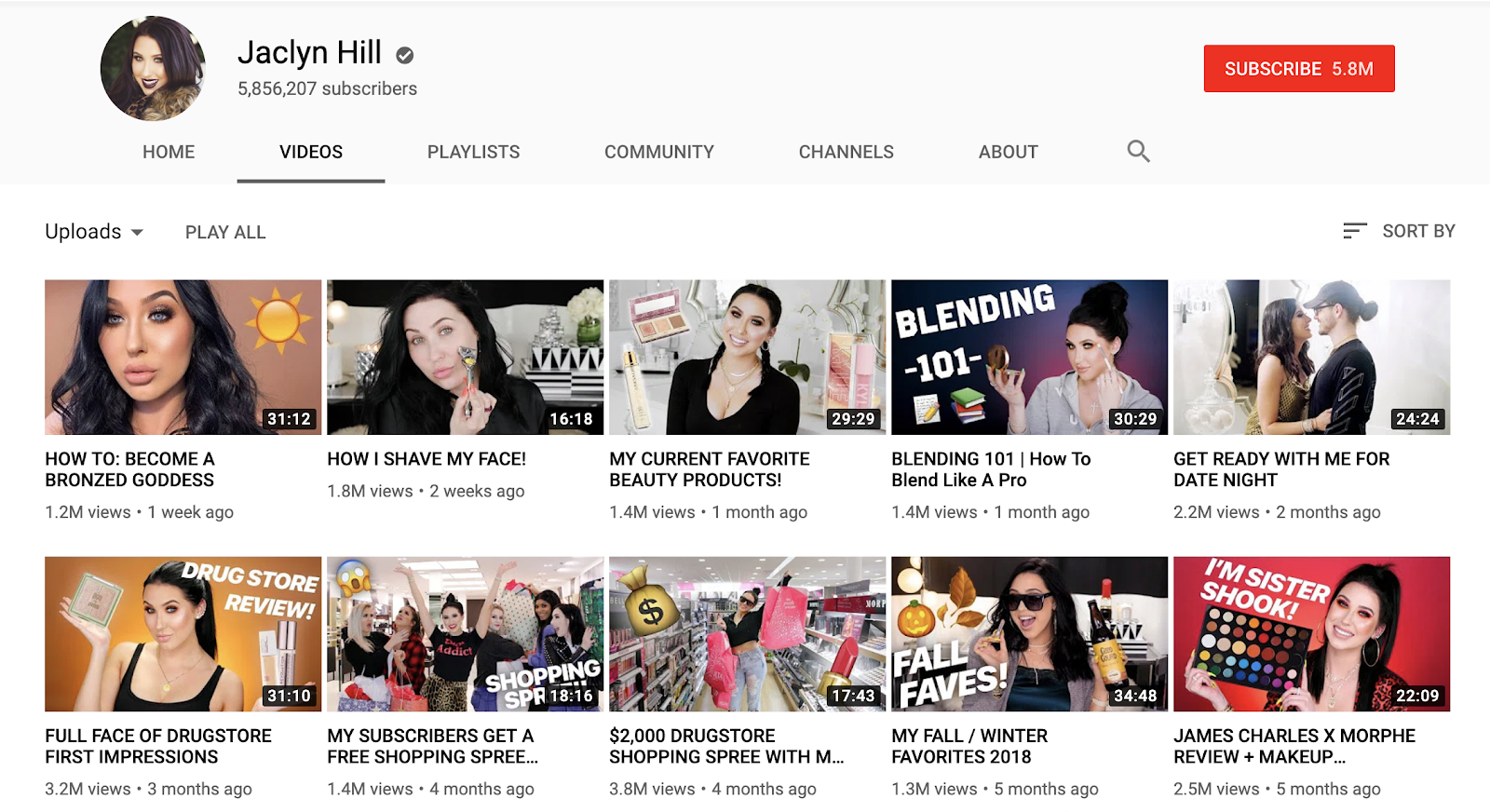The image is a detailed screenshot of the YouTube channel of Jacqueline Hill. In the top left corner, there is a circular profile icon featuring a woman with long, dark hair. Adjacent to it is the channel's title, "Jacqueline Hill," which has an impressive subscriber count of 5,856,207. On the top right, there is a prominent red "Subscribe" button displaying "5.8M" subscribers.

Below the profile photo and channel name are various clickable tabs including Home, Videos, Playlists, Community, Channels, About, and a Search icon. The "Videos" tab is currently selected, offering options to view Uploads, Play All, and Sort By.

The main content area displays two rows of video thumbnails, each row containing five videos. Each thumbnail features the same woman and shows the video's length. Underneath each thumbnail, the video's title, view count, and posting date are listed.

The titles of the videos in the top row from left to right are:
1. "How to Become a Bronzed Goddess"
2. "How I Shave My Face"
3. "My Current Favorite Beauty Products"
4. "Blending 101: How to Blend Like a Pro"
5. "Get Ready With Me for a Date Night"

In the second row, the video titles include:
1. "Full Face of Drugstore First Impressions"
2. "My Subscribers Get a Free Shopping Spree"
3. "$2000 Drugstore Shopping Spree with..."

Further details of the last video in the second row are not visible in the screenshot.